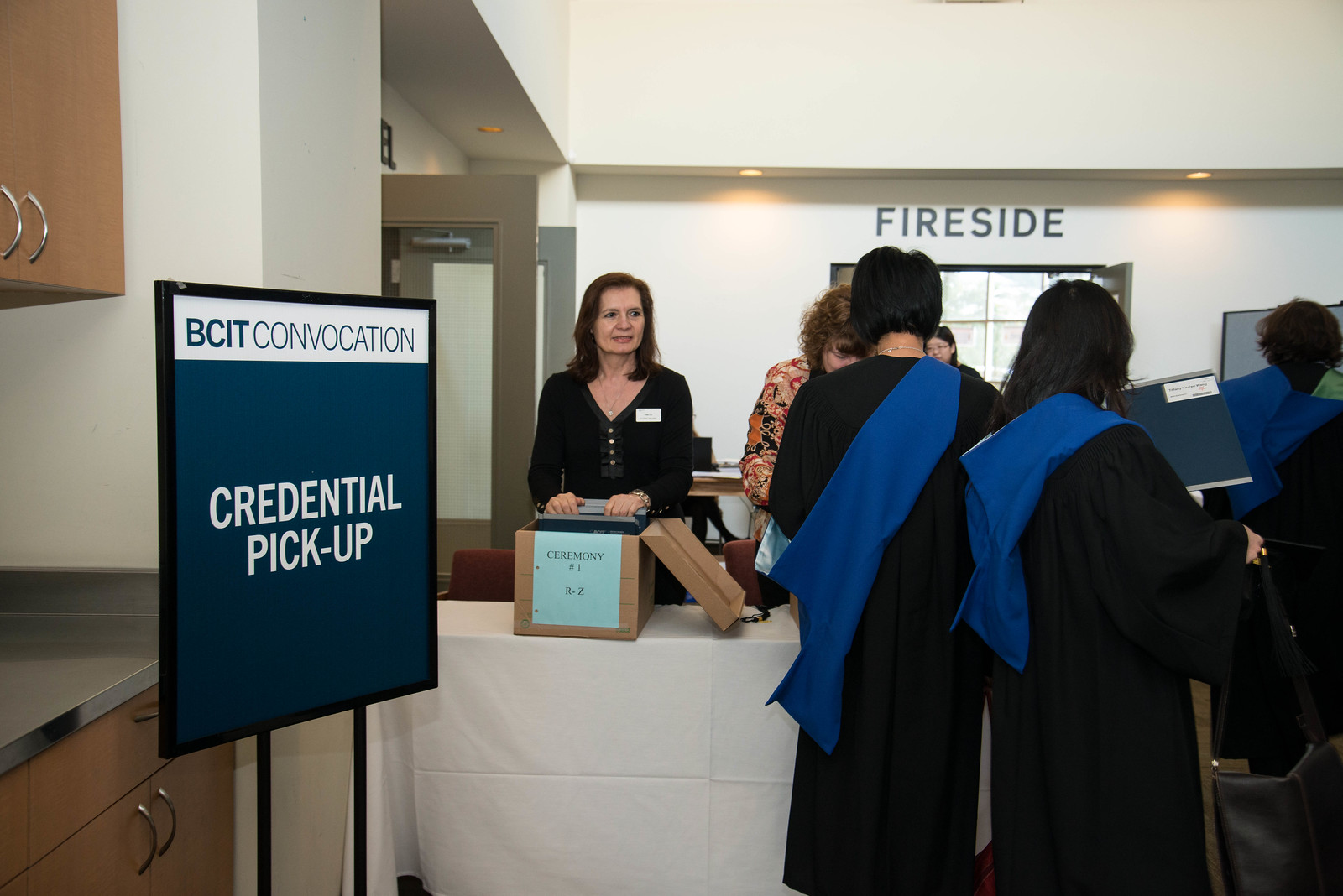This detailed photograph captures a post-graduation convocation scene, likely at BCIT. Central to the image are two women, clad in black graduation gowns and blue sashes, standing back-to-back and facing a folding table draped in a white tablecloth. Behind this table are several older women; one is handling a cardboard box labeled "Ceremony: R to Z," which has a blue paper affixed to it. Prominently displayed to the left of the table is a sign that reads "BCIT Convocation Credential Pickup," indicating the women in gowns are retrieving their diplomas or credentials. One of the graduates holds a blue binder with an indistinguishable white label. Further along in the background, other individuals wearing similar graduation attire suggest a gathering of graduates collecting their ceremony credentials. The indoor setting is brightly lit, with colors such as brown, white, dark blue, black, light blue, maroon, gray, silver, and orange visible throughout the scene. A door marked "Fireside" stands open in the background, reinforcing the indoor and likely daytime setting.